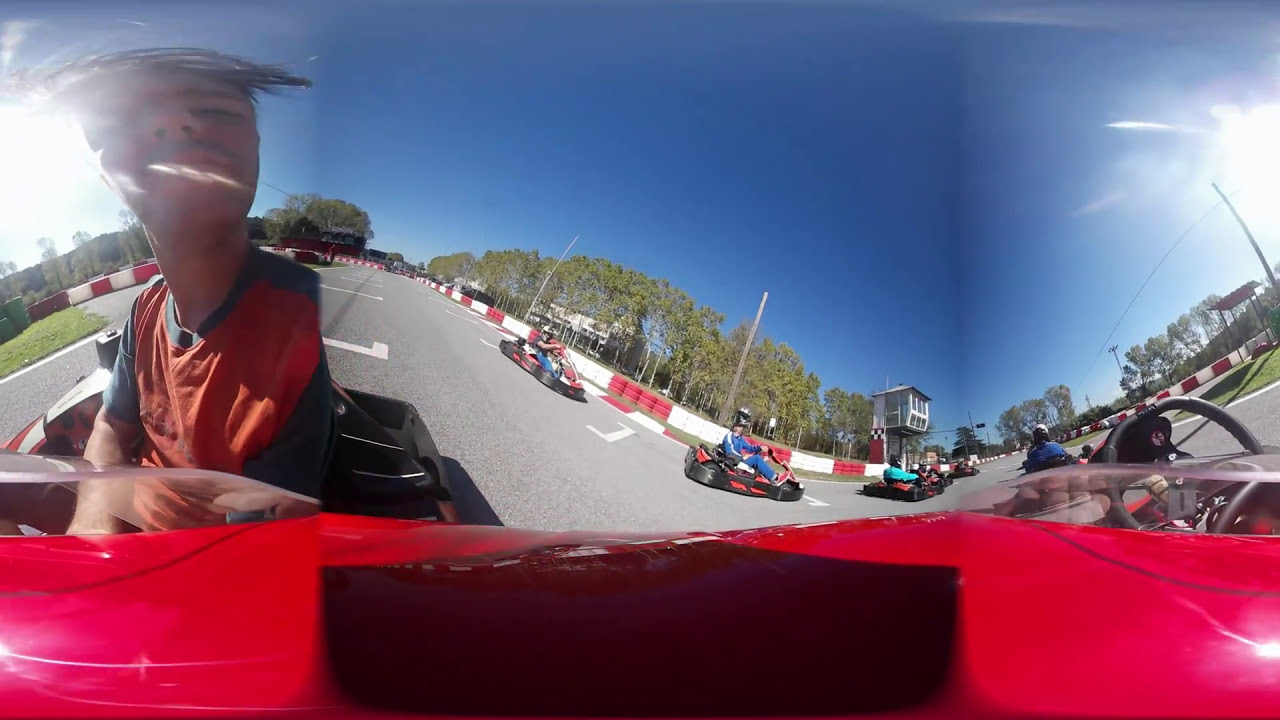This is a highly detailed, panoramic 360-degree image capturing a vibrant bumper car ride on a large asphalt lot. In the immediate foreground, there is a hot pink neon bumper car with a young teenage boy at the wheel. His dark hair is windswept, and he has a five o'clock shadow. He is wearing an orange and blue-gray t-shirt. The scene is vividly sunlit, casting well-defined shadows, and the sky is a brilliant, cloudless blue. Surrounding the lot is a guardrail made of red and white tires. Outside the guardrail, you can see tall trees stretching along the horizon and an observation tower elevated on stilts. Positioned on the left, the partially visible Sun adds a glowing hue to the scene. The image's 360-degree nature creates some warping and blurriness, particularly noticeable around the edges. Scattered throughout the lot are numerous other brightly colored bumper cars with riders, some wearing helmets, adding to the lively energy of the scene.